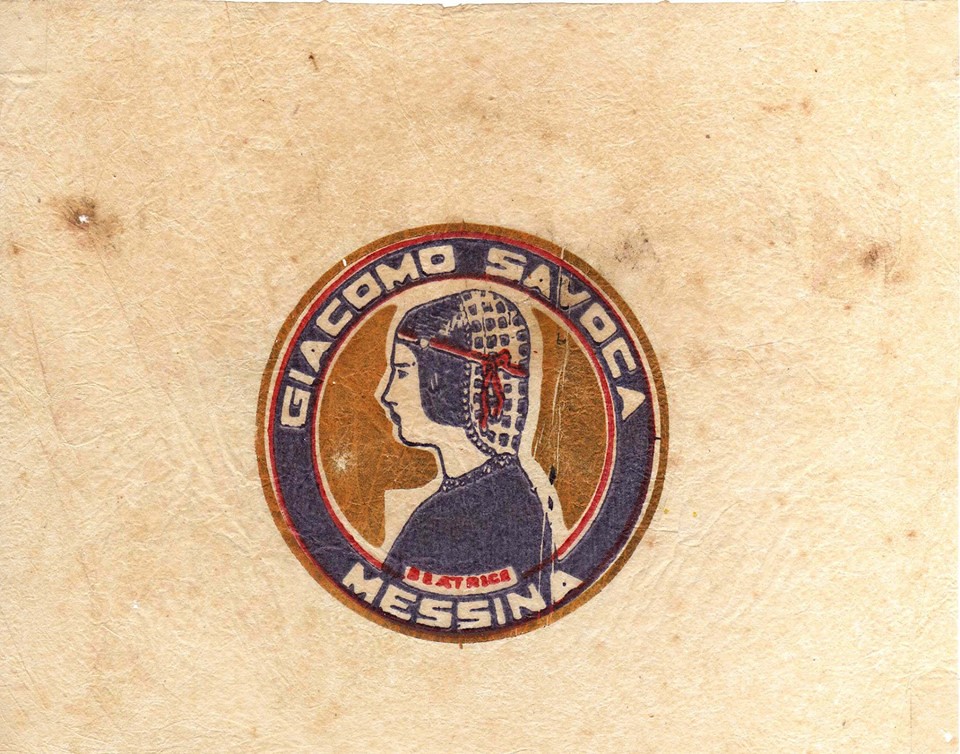The image depicts a seal centered on a weathered, cream-colored parchment with dark blotches of discoloration, giving it an antique appearance. The seal itself features a circular design with a brownish-yellow border encircling a blue band. The blue band bears white lettering that reads "Giacomo Savoca" at the top and "Messina" at the bottom. Within the innermost circle, which shares the brownish-yellow color of the outer border, there is a detailed illustration of a woman. She has pale skin and is adorned with a checked headscarf of white and blue, tied with a red bow. The woman also wears a blue shirt. The intricate and vivid details of the seal contrast sharply with the rustic texture of the parchment, creating a striking visual juxtaposition.